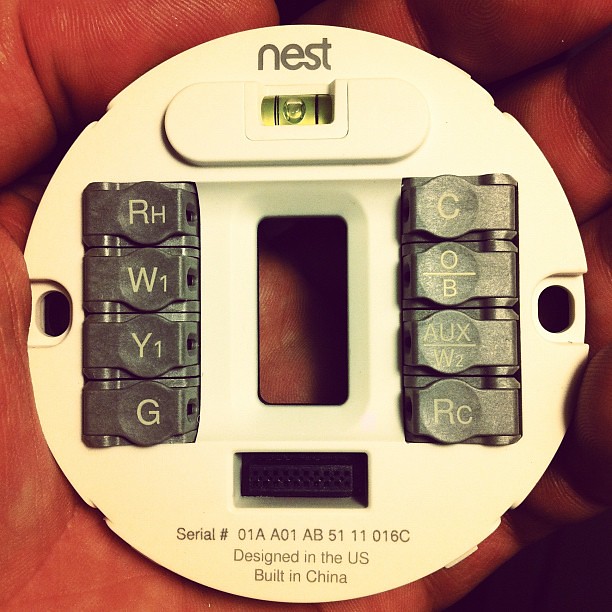This image is a close-up, macro photograph showcasing a Nest thermostat base held in someone's hand. The base is predominantly white with a circular design. At the top of the circle, the word "Nest" is clearly visible, indicating the brand. Below the Nest logo, there appears to be a small light or sensor. Flanking the center are two holes, possibly for mounting screws, and in the middle, there is a large rectangular slot, which could be for wiring or other connections.

To the left and right of this slot are two vertical columns of black buttons or terminals. In the left column, from top to bottom, the labels on the buttons read: "RH," "W1," "Y1," and "G." In the right column, the labels read: "C," "O/B," "AUX/W2," and "RC," with a line separating some of the labels. 

At the bottom of the circular base is a smaller rectangular slot with several holes, likely for additional connections or plug-ins. Engraved or printed below this slot is a serial number: "01AA01AB511100016C," accompanied by the text "Designed in the U.S." and "Built in China." This detailed and intricate description suggests a component used for smart home heating and cooling control systems.